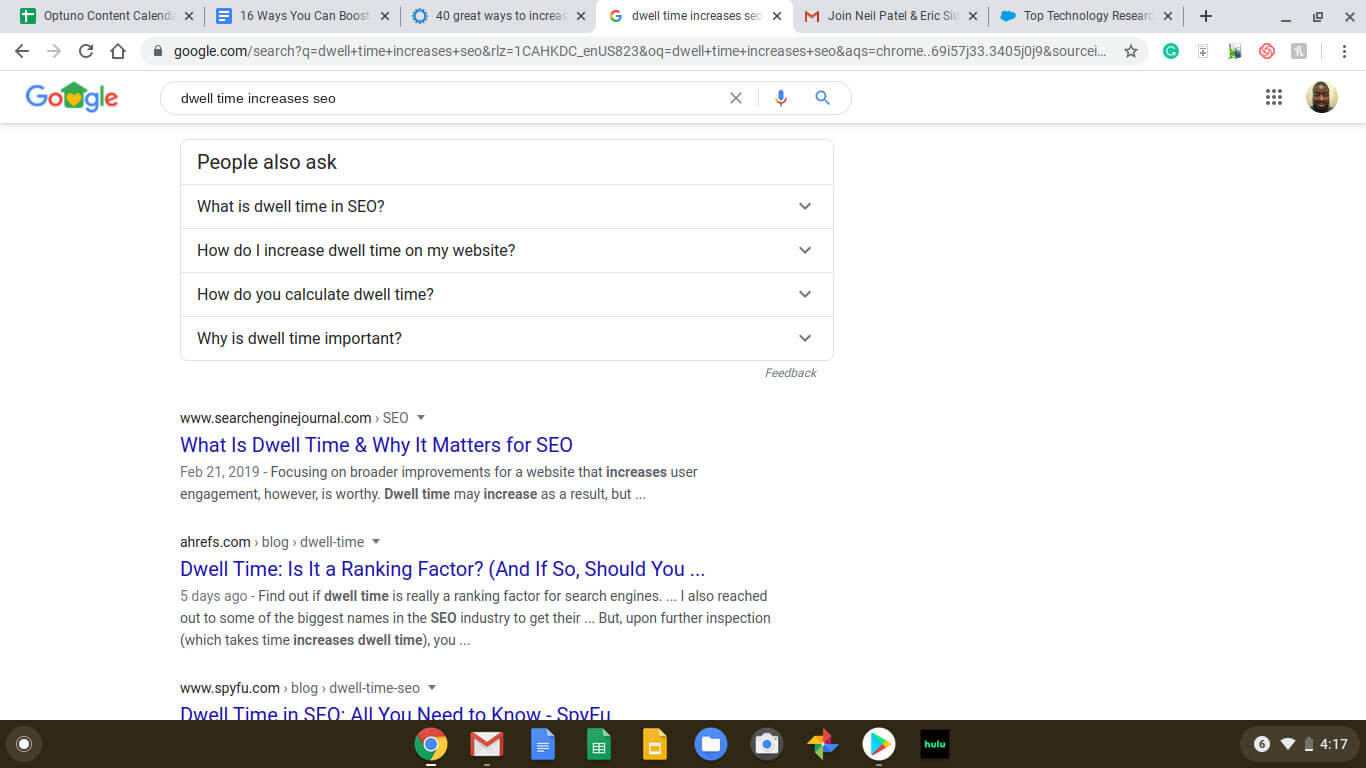The image depicts a large, colorful Google search page. The iconic Google logo is prominently displayed at the top, with individual letters in blue, red, yellow, blue, and green, and the letter "E" in red. Below the search bar, someone has typed the phrase "dwell time increases."

The search results reveal a segment commonly labeled as "People Also Ask," featuring questions such as "What is dwell time in SEO?" and "How do I increase dwell time on my website?" Sequentially, other queries include "How do you calculate dwell time?" and "Why is dwell time important?" 

Following the questions are article links, the first titled "What is dwell time and why it matters for SEO," accompanied by a brief description in black text. Another article titled "Dwell time: Is it a ranking factor?" appears in purple text, indicating it has been visited. This article was posted five days ago and elaborates on the significance of dwell time as a ranking factor. Further down, another article titled "Dwell time in SEO: All you need to know" is partly visible, with the bottom portion truncated and showing only partially readable text.

At the bottom of the screen, there is a black strip containing the usual computer icons and menu options, completing the typical layout of a search engine results page.